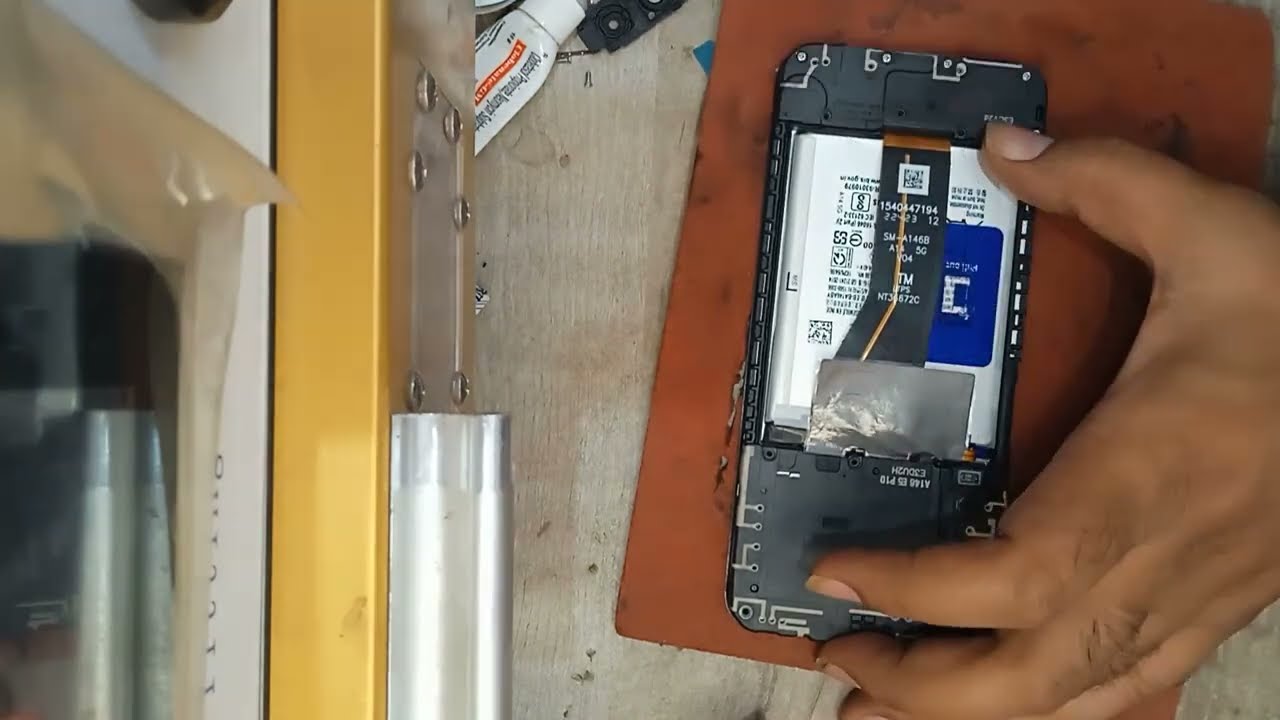The photograph captures a meticulous scene of someone working on disassembling a smartphone from an overhead perspective. The primary focus is on a dark-skinned hand with dirty fingernails gripping an upside-down cell phone with its back panel removed, revealing an exposed battery marked with a white label and blue tab, and a piece of duct tape securing it alongside a visible copper wire. The phone rests on a rectangular brown placemat atop a light, raw, unfinished wooden tabletop. Close by, a white tube with black and red text, possibly glue or ointment, lies with its cap on. Further to the left, yellow cabinet drawers with silver handles are visible, with a black and silver rectangular object in a plastic bag placed atop them. Additionally, a beige metal piece is vaguely discernible in the frame. The surroundings suggest a workshop-like environment, given the presence of various tools and repair parts, encapsulating a hands-on and detailed moment of electronic repair.